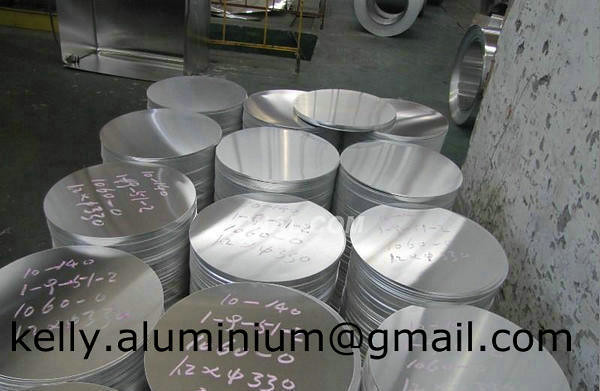The image features twelve stacks of circular aluminum sheets, meticulously cut and stacked in three columns and four rows. Each stack is marked with various white numbers. At the bottom of the image, the email address "kelly.aluminium@gmail.com" is printed in black. The setting appears to be a gray, concrete-floored warehouse or workspace. To the right stands a white wall, and in the top left corner, an aluminum box is positioned near a yellow metal fence, reinforcing the organized yet industrial essence of the scene.